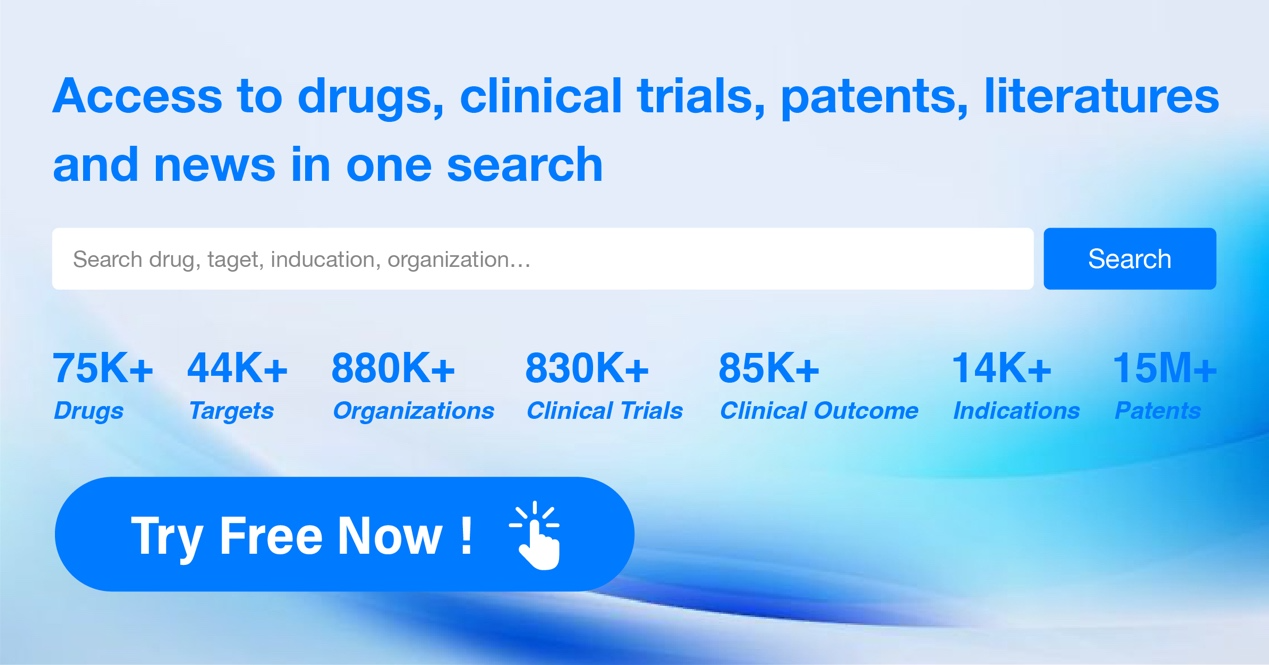A detailed screenshot of a website showcases a comprehensive search engine designed for medical professionals. The site boasts the ability to access drugs, clinical trials, patients, literature, and news through a single search interface. The central focus is a white search bar with black lettering, positioned prominently against a blue-toned background that graduates from light blue at the top to a deeper blue, swirling downward at the bottom.

Key figures highlighted in blue text include: 
- 775,000+ drugs
- 44,000+ targets
- 880,000+ organizations
- 830,000+ clinical trials
- 85,000+ client outcomes
- 14,000+ indications
- 15 million+ patients

A call-to-action "Try Free Now" stands out in white text. The layout is designed to be user-friendly and visually appealing, emphasizing the breadth of information available through the platform.